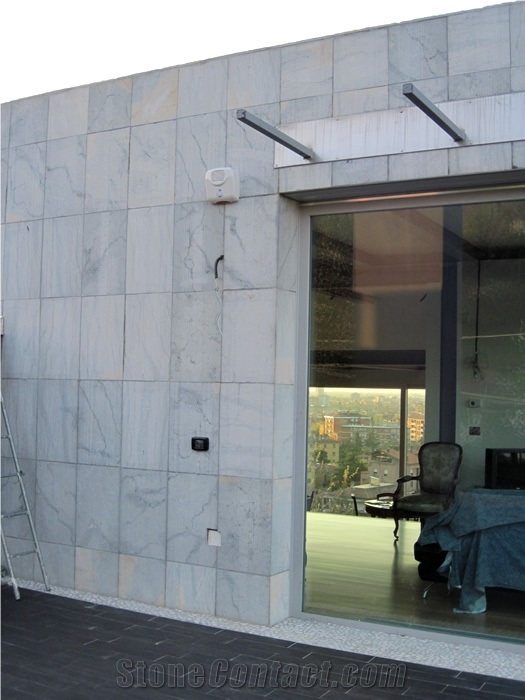The image showcases the exterior of a square, minimalist, high-end building, likely an apartment or small residence, featuring light gray stone tiles reminiscent of marble. The left half of the image is dominated by this stone facade, with a partial view of a ladder and what seems to be an outdoor outlet and a security system. In the lower section, a watermark reading "stonecontact.com" suggests that this could be a reference image for a stone contractor's portfolio.

Centered is a large, floor-to-ceiling window or perhaps a window panel section, bordered by protruding metal beams and a PA speaker in the upper left corner. Through the glass, the interior of a modern room unfolds, revealing a wooden floor and a table draped with a blue cloth or tarp. An upholstered wooden chair is also visible. On the far end of the room, another sizeable floor-to-ceiling window frames a cityscape with other residential buildings in the distance. The interior appears to be well-lit, emphasizing its airy and open design.